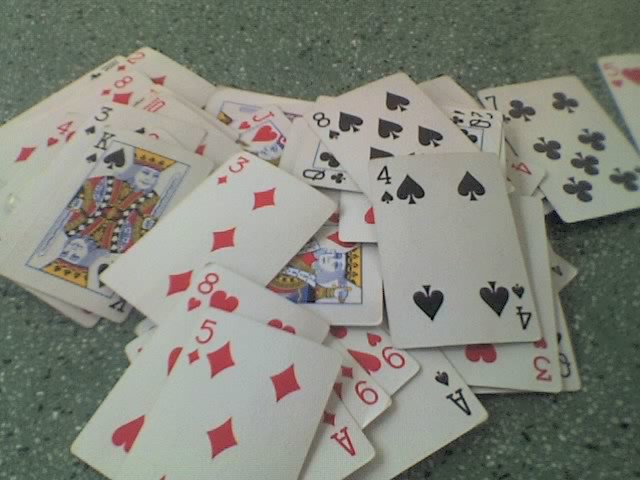In this image, a scattered deck of playing cards is sprawled chaotically across a smooth, green particleboard table. Among the visible cards, we spot the five of diamonds, eight of hearts, three of diamonds, ace of diamonds, and ace of spades. A full four of spades card is apparent, with part of an eight of spades partially visible beneath it. Further down, there’s a hint of the queen of clubs. The collection includes a king card, likely the king of hearts, while most of the king of spades can be seen on the left side. The spread also reveals a three of spades, as well as the ten and eight of diamonds. In the image's lower right corner, the seven of clubs is almost completely visible, with just the edge of the five of hearts next to it. Overall, the scene depicts a full deck of cards haphazardly strewn across the table, with some cards more discernible than others.